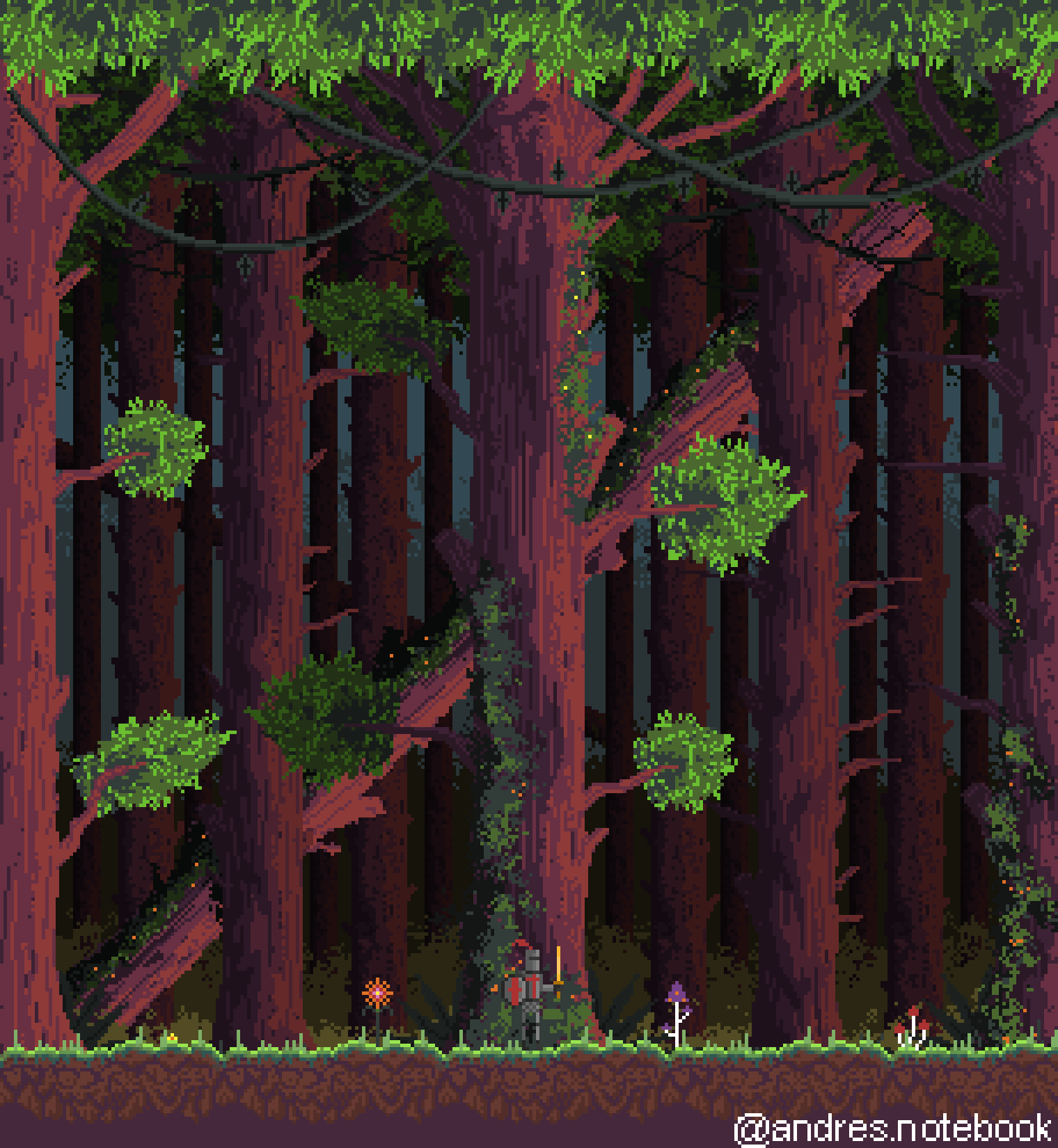In this pixelated side-scrolling game image, the setting is a dense forest reminiscent of a Redwood grove. The forest floor is layered with a thin strip of vibrant green grass atop a substrate of earthy soil, much like the style of Terraria. Towering, ancient trees dominate the scene, their massive trunks stretching upward. The looming canopy above is a mix of brilliant green foliage and gnarled branches. In contrast, the background trees gradually diminish in size and darken in color, creating an atmospheric depth that evokes the twilight of dusk.

Lush vegetation abounds with mushrooms and various flowers dotting the forest floor. The overall scene is shadowy, suggesting the edge of the forest, where light still penetrates, as opposed to the impenetrable darkness within. The sky is a muted gray, adding to the dusky ambiance.

In the foreground, there are four brightly highlighted trees with prominent tufts of leaves. Among them lies a fallen tree, partially obscured but adding to the depth and mystery of the forest. The hero of the game stands prominently in the middle of the image. This character is a knight clad in dark armor accented with red details. They wear a distinct kettle helmet adorned with a striking red feather. The knight wields a golden sword, possibly magical in nature, poised and ready for adventure.